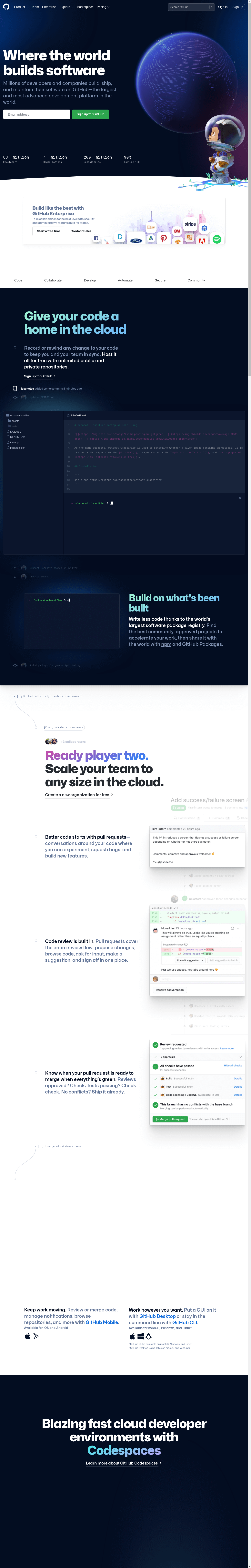A visually complex image featuring a detailed, multi-element design. The top portion of the image has a solid black background with white text. Below that, there's a small box with a gradient from white to green. Dominating the central area, a large, oblong blue shape is prominently displayed. Within this shape, there's a small figure resembling a spaceman. To the right, there's a white block containing blue text and multiple colored elements in blue, red, and green.

Further down, a large, dark blue box occupies a significant portion of the image, featuring light blueprints at both the top left and bottom right corners. Adjacent to this is a white box bordered by a blue outline, also featuring blueprints. Inside this white box are several smaller white boxes outlined with green lines.

The bottom of the image reverts to a black background with white text, and there are blue elements at the very bottom. The text in this area is very small and difficult to read.